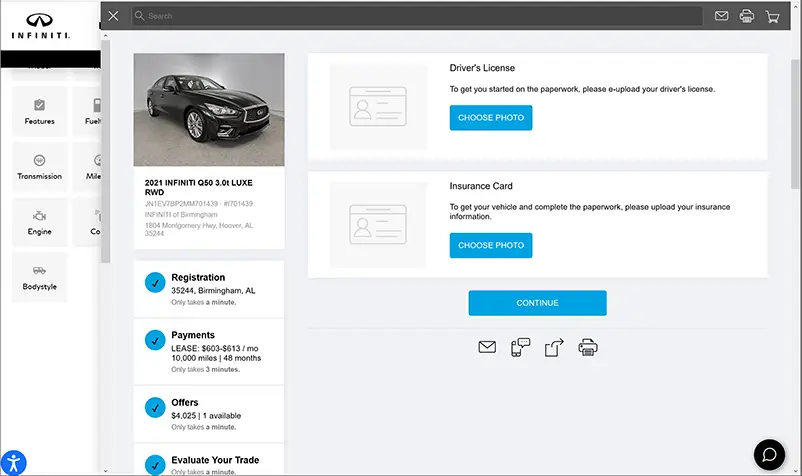Screenshot Description:

The screenshot features a user interface with multiple sections. On the left-hand side, less than an eighth of the way in, a white background showcases black text. Above the text is a graphic resembling an upside-down Pac-Man or a pizza with a slice taken out, accompanied by the word "INFINITI" in black.

Beneath this, the white background continues with gray squares containing black text. These squares list categories such as "Features," "Transmission," "Engine," and "Body Style" in a vertical arrangement. Adjacent to "Features" is a square labeled "Fuel," next to "Transmission" is the word "Mile," and beside "Engine" is the abbreviation "CL."

On the right-hand portion of the screenshot, another interface overlays the previous one, featuring a black background. In the upper right-hand corner, there are white icons for search, email, printer, and a shopping cart. This section has a light grayish background and displays a black car within a showroom-like setting.

The main text in this section reads "2021 INFINITI Q50 3.0T LUX RWD" in black, along with VIN numbers and additional details in gray. It also includes registration information and lease payment options, indicating rates between $306,000 to $316,000 per month. Additional fields are present for entering a driver's license and insurance information, presumably for leasing the car.